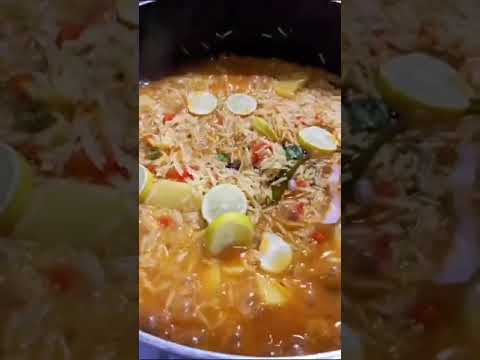This wide rectangular image is divided into three parts: a central tall vertical photograph showing the contents of a cooking pot, flanked by narrow rectangular close-up shots of portions of the main image. The central photograph reveals a pot, partially visible at the top and bottom edges, containing an orange-colored liquid soup. Floating in the soup is a mix of thick, beige-colored noodles and various vegetables. Dominating the mixture are circular yellow slices, possibly zucchini or lemon, scattered throughout. Additionally, there are red and green vegetables, potentially tomatoes or peppers, adding vibrant color. The close-up sections on the sides focus on these details, showing a variety of ingredients, including shredded or thin components that resemble either cabbage or cheese, and enhancing the overall visual of the soup's rich texture and diverse ingredients. The pot adds a gray, curved frame at the top and bottom, with the top part appearing darker. The entire setup is brightly lit, especially in the central photograph, bringing out the intricate details and colors of the soup.